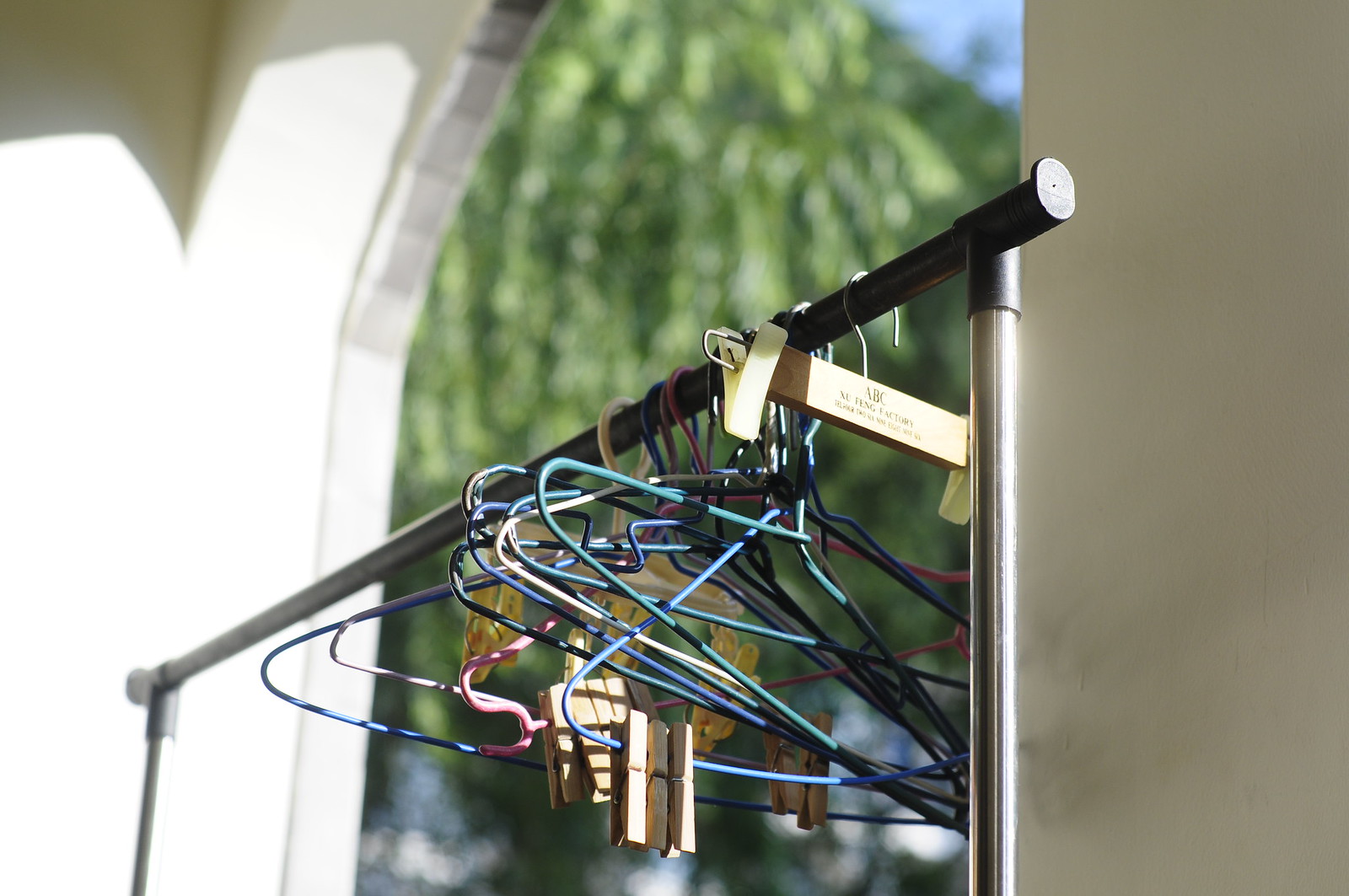This image captures an outdoor scene viewed from within an arched doorway next to a white wall. Through the open door, a vivid blue sky and a lush green tree are visible, providing a serene backdrop. Inside the doorway, there is a black clothes rack with a sturdy steel frame, likely mobile though only the top half is visible. The rack supports around 15 varied hangers, ranging in color from blue, pink, purple, and black, to brown. Among these, a distinct wooden baby hanger contrasts with the more common metallic hangers. Some hangers are affixed with clothes pins, colored pixels—a detail with several hangers showing between 2 to 5 small pixels, presumably decorative or functional marks. The overall composition of the photo emphasizes a juxtaposition of vibrant, diverse hangers against the calming natural scenery outside.